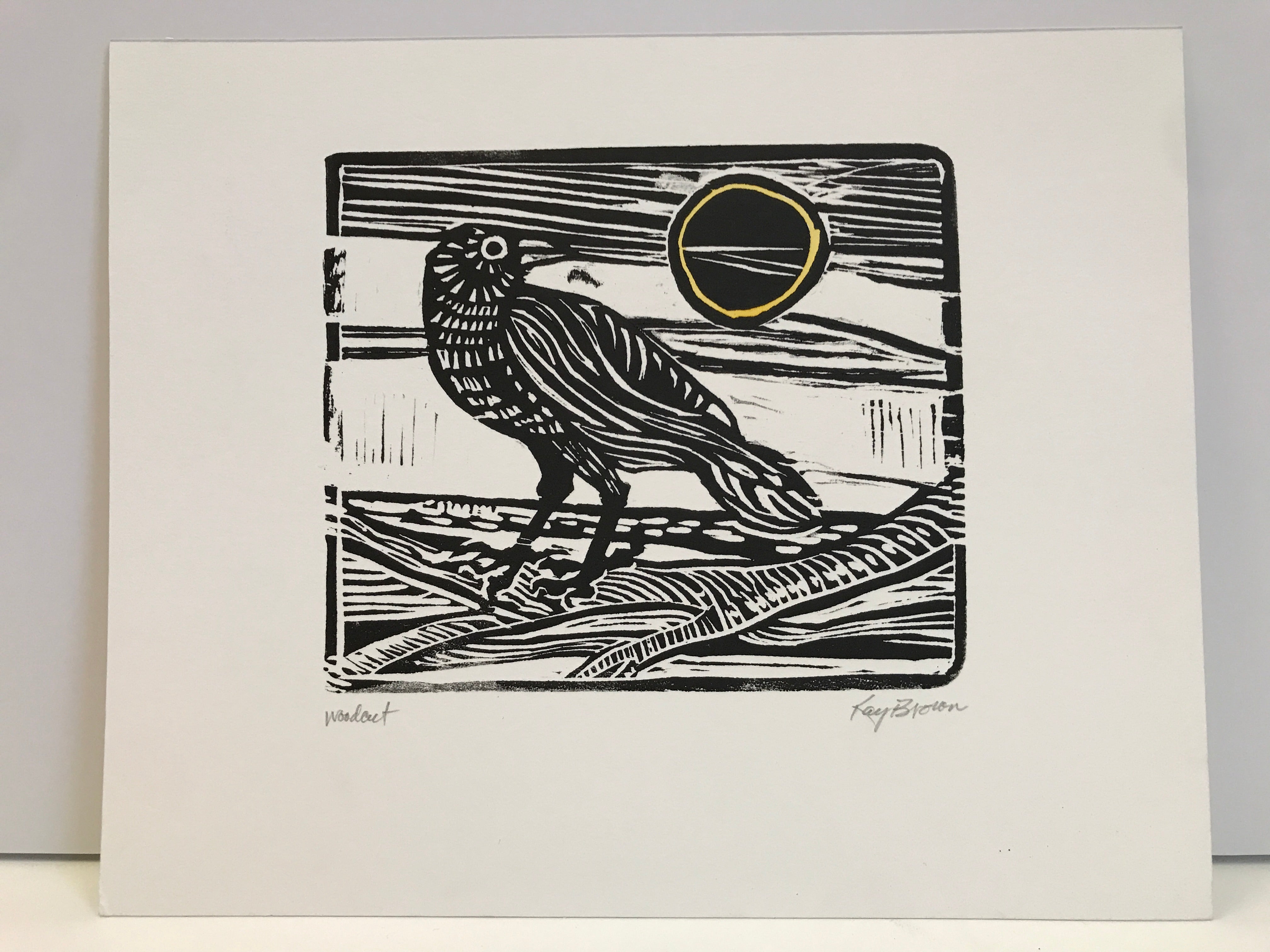The image depicts a rectangular, black-and-white drawing with an off-white background and a gray outer frame. Central to the piece is a bird resembling a crow or blackbird, perched on a tree branch. The bird, situated in a square in the middle of the drawing, faces left while looking back over its shoulder to the right, towards a black circle with a yellow outline, suggesting an eclipse or the sun. The sky around the bird and the circle is marked with black streaks, enhancing the contrast. The bottom left and right corners of the image feature indecipherable signatures, possibly reading as Ray Blunden or K. Brenton. The artwork bears a handmade quality, reminiscent of ink or paint stamped onto cardstock.